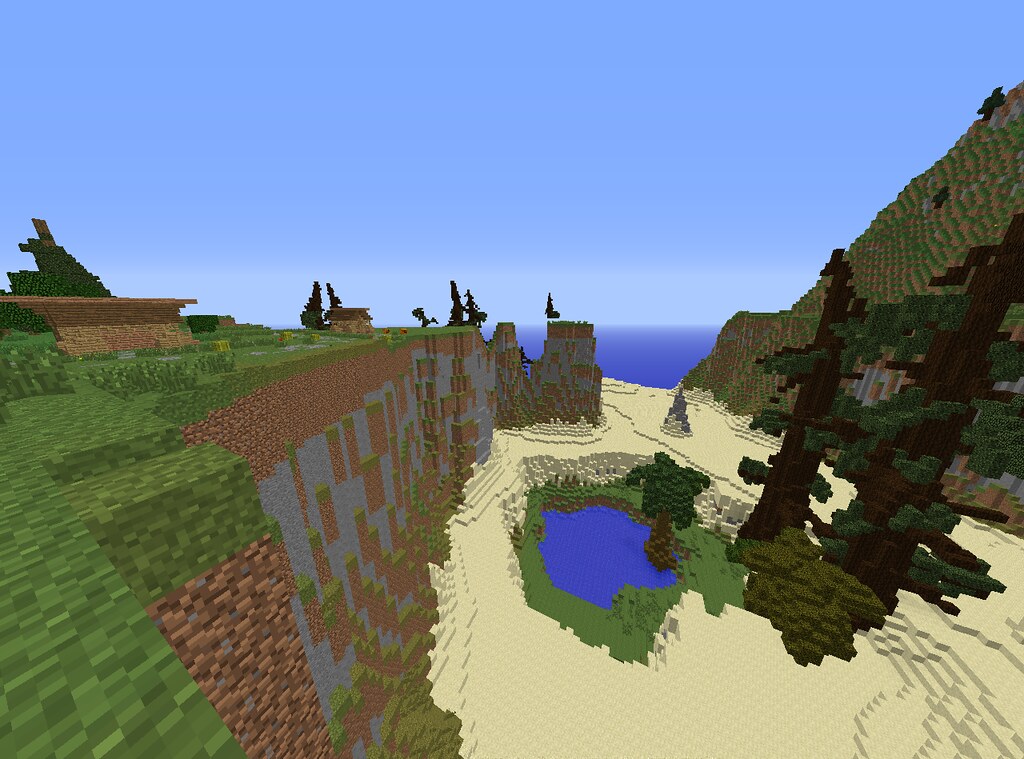This Minecraft screenshot captures a vibrant, blocky landscape. On the left, a tall cliff composed of pixelated grass and dirt rises prominently. Below, pixelated sand or dirt stretches across the ground, leading to a small, serene stream flowing through the center of the image. Surrounding this water feature are tall trees with blocky, pixelated leaves. To the right, another imposing hill or mountain ascends, its summit cloaked in lush green grass. The sky above is a clear blue, offering a peaceful backdrop, while an ocean's expanse is visible in the distant horizon. Atop the left cliff stands a structure resembling brickwork, accompanied by pixelated bushes to its side and a pixelated tree directly behind, adding a rustic touch to this picturesque Minecraft scene.